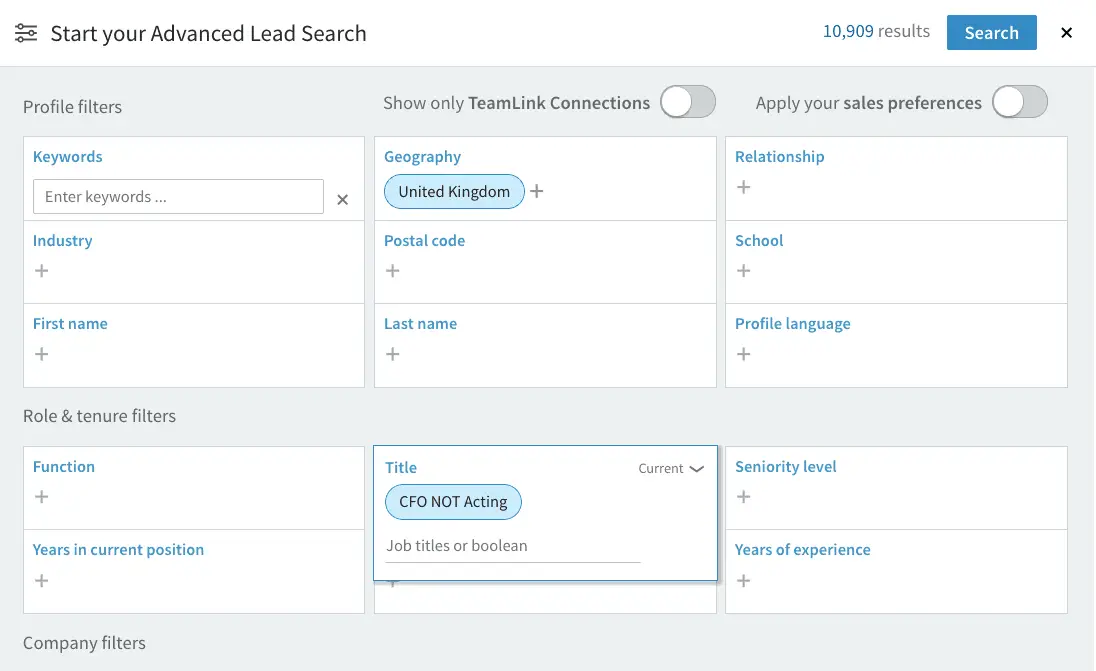The screenshot showcases an advanced search interface on a sales platform. At the top left corner, the title "Start Your Advanced Lead Search" is prominently displayed. The top right corner shows "10,909 results," indicating the number of matches. Below this, there's a prominent blue "Search" button.

Directly underneath the search button, there is a grey box labeled "Profile Filters," with fields for entering "Keywords," "Industry," and "First Name." Adjacent to this, the interface includes additional options like "Geography," where "United Kingdom" is highlighted in a blue oval. Further options below include "Postal Code," "Last Name," "Relationship," "School," and "Profile Language."

At the top, two toggle sliders are displayed: "Show Only Team Link Connections" and "Apply Your Sales Preferences," both currently in the 'off' position.

The bottom section is labeled "Role and Tenure Filters," featuring multiple options such as "Function and Years in Current Position," "Title," and specific job roles. For instance, there's a blue pill-shaped button labeled "CFO (current)" and beneath it, an input field for "Job Titles or Billions." To the right, there are fields for "Seniority Level" and "Years of Experience," offering comprehensive filtering options for targeted lead searches.